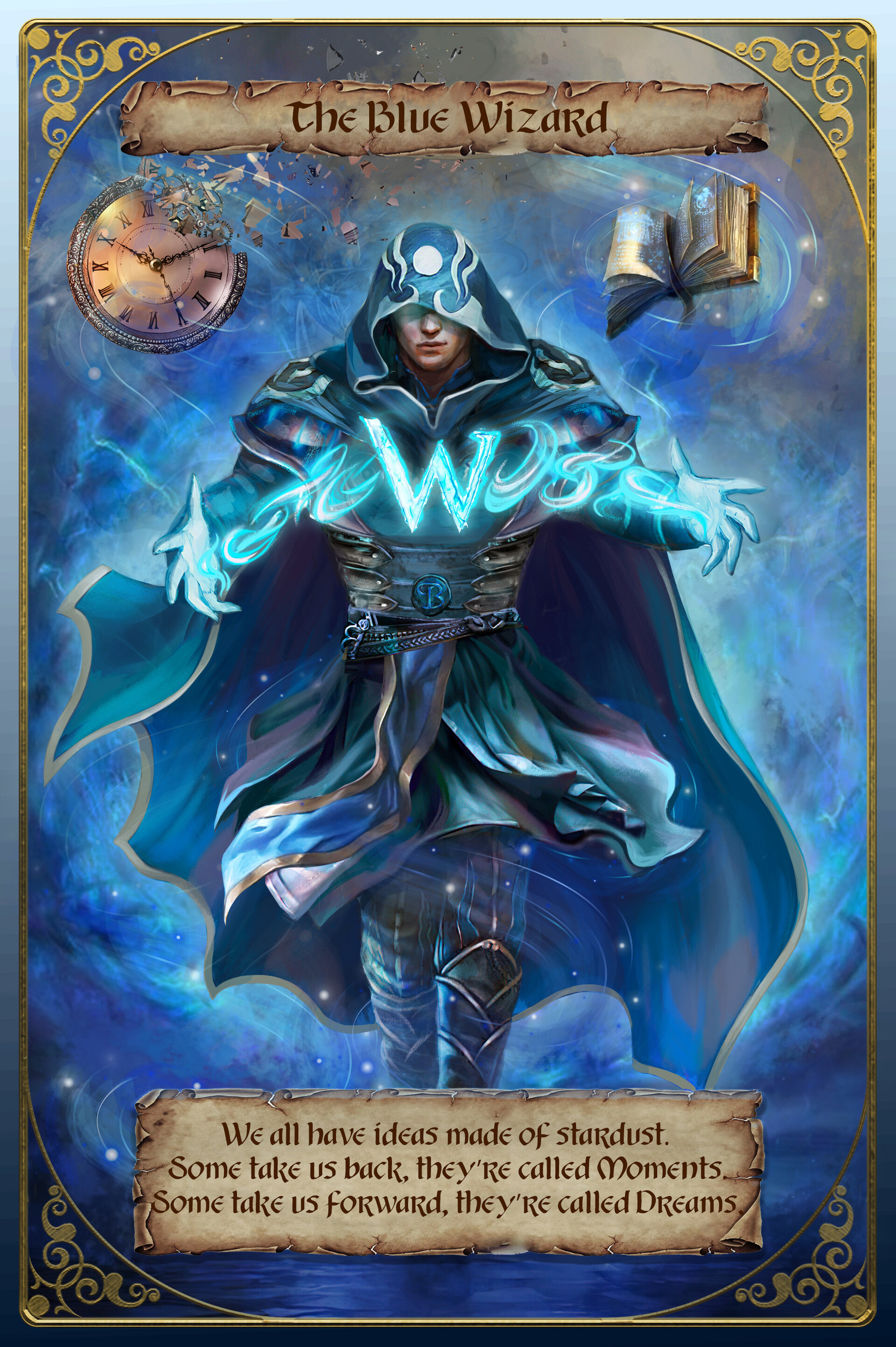This vertically-oriented fantasy image, resembling a trading or playing card, prominently features "The Blue Wizard" in bold, dark brown medieval font on papery-looking text boxes at both the top and bottom. The centered figure, a white man in his 20s or 30s, is cloaked in a bright blue, heavy robe that obscures most of his body and face, leaving only his nose and mouth visible. His unique attire includes a belt with the letter 'B' and chest markings that might be part of an incantation, highlighted by a glowing 'W' between his hands as he chants or casts a spell. The background is a blue, swirling mist, adorned with a deteriorating clock in the top left and a spellbook in the top right, all bordered by intricate gold engravings. The bottom text box holds an inspirational message: "We all have ideas made of stardust. Some take us back, they're called moments. Some take us forward, they're called dreams." The artistic layout invokes the feel of a magical, animated tarot card brought to life.